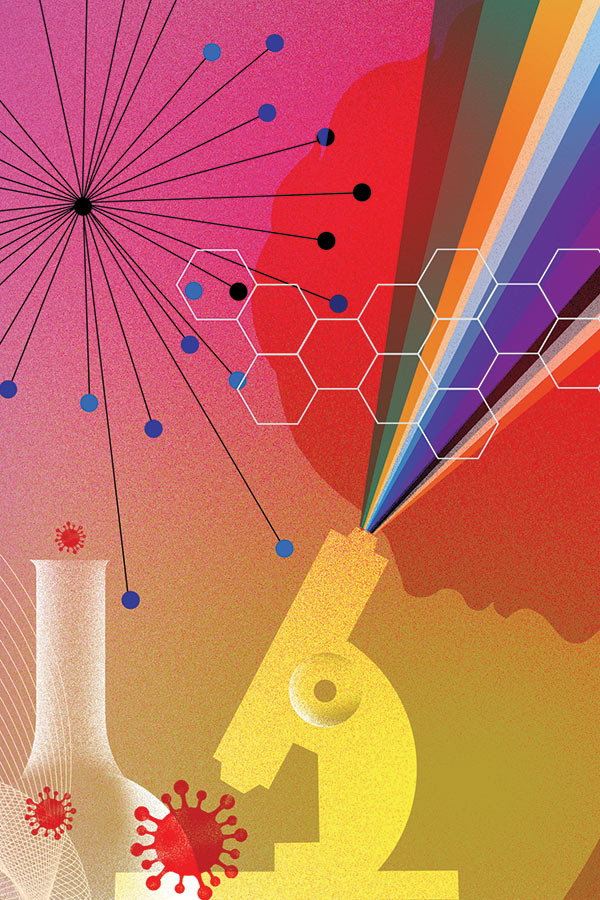In this computer-generated image with a pink to light yellow, glittery, and pixelated background, a yellow microscope is prominently featured in the lower center, tilting from left to right. Vibrant beams of red, orange, yellow, green, blue, light blue, purple, pink, and red shoot out from its top, resembling a spray of rainbow colors. To the left of the microscope, a white, frosty-colored laboratory beaker with a long neck and round body stands. Surrounding the beaker and microscope are multiple red virus-like shapes with tentacle-like extensions ending in circles. In the upper right corner, a striking black circle features several black lines extending in all directions, tipped with blue circles. Across the middle right of the image, a white hexagonal grid pattern is visible, adding a scientific, chemical compound appearance to the artwork. Overall, the image evokes a sense of scientific exploration through its abstract and colorful elements.